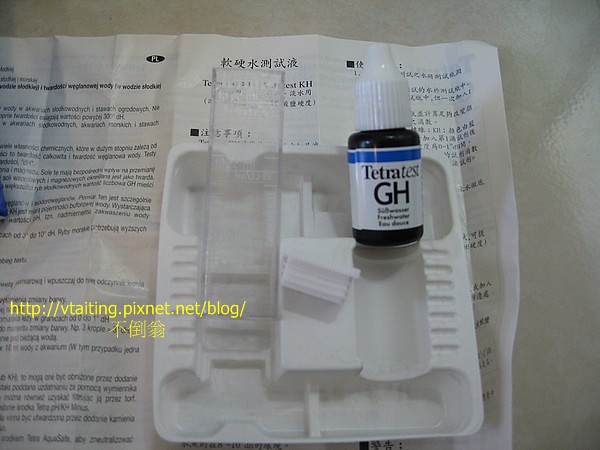This photographic image prominently features a small, dark brown bottle with a white twist-off cap labeled “T.E.T.R.A. test G.H. Freshwater” in black text, and a blue stripe at the top of the label. The bottle, which resembles medication or a medical supply like eyedrops, sits on a white plastic tray. This tray is placed atop an open brochure. The brochure contains text in multiple languages including a page with Asian characters and another that appears to be in German or French, though the text is too blurry to discern clearly. On the left side of the brochure, there is a section with yellow lettering that includes the website “http://vtaiping.pixnet.net/blog/” followed by several Asian characters. No people are visible in this image. The predominant colors are gray, blue, white, and yellow. The background of the photo is light gray.